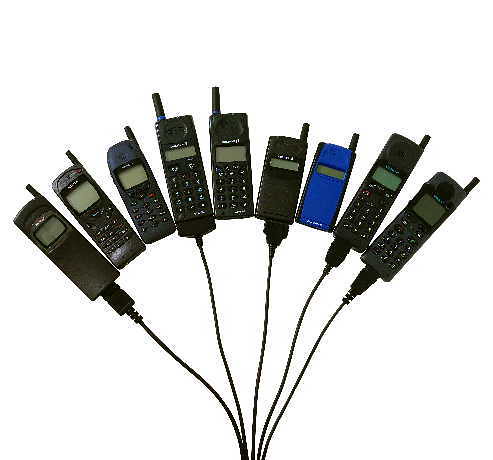This pixelated photograph features a collection of nine vintage cell phones arranged in a half-circle, reminiscent of a setting sun. Dating back to the late 1990s or early 2000s, these large, clunky phones are equipped with visible antennas and old-fashioned LCD displays, likely only capable of showing basic information like phone numbers. Most of the phones are black, with a notable blue one among them. Five of the phones are connected to a variety of power cords, which differ from the standardized charging methods we use today. Several of the devices appear to be flip phones with keypads potentially covered. All the phones exhibit some small text on their displays, though it's indistinguishable due to the pixelation of the image.